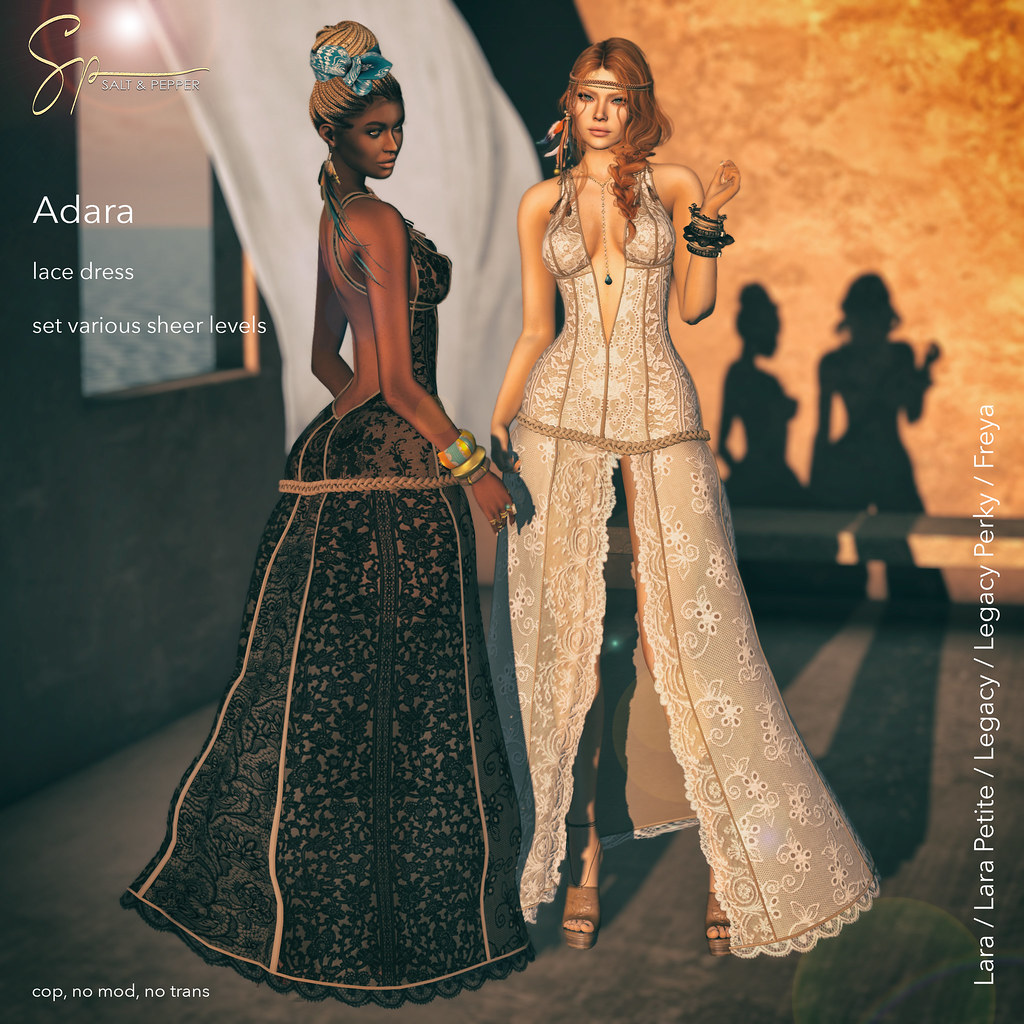The 3D animated image features two intricately detailed women positioned centrally as part of what appears to be a fashion advertisement. At the top left corner, the text reads "Salt and Pepper," followed by "Adara" and "Lace Dress, Set Sheer Levels." Further down on the lower left, phrases like "Cop, No Mod, No Trans" are visible. 

On the right side of the image, starting from the bottom corner and ascending vertically, the text includes "Lara, Lara Petit, Legacy, Legacy Perky, Freya." 

The left woman has dark skin and wears a black lace dress. Her black hair, braided and tipped with blonde, is styled up into a bun secured with a bandana featuring a blue bow. She accessorizes with multiple colorful bracelets on her right arm. 

The right woman, with fair skin and reddish hair, dons a white lace dress with a plunging neckline that extends to her belly. A headband adorned with dangling feathers wraps around her forehead. She also wears a statement necklace and several bracelets on her right arm.

The overall aesthetics and detailing of the characters suggest an advertisement-like quality aimed at promoting fashionable garments.